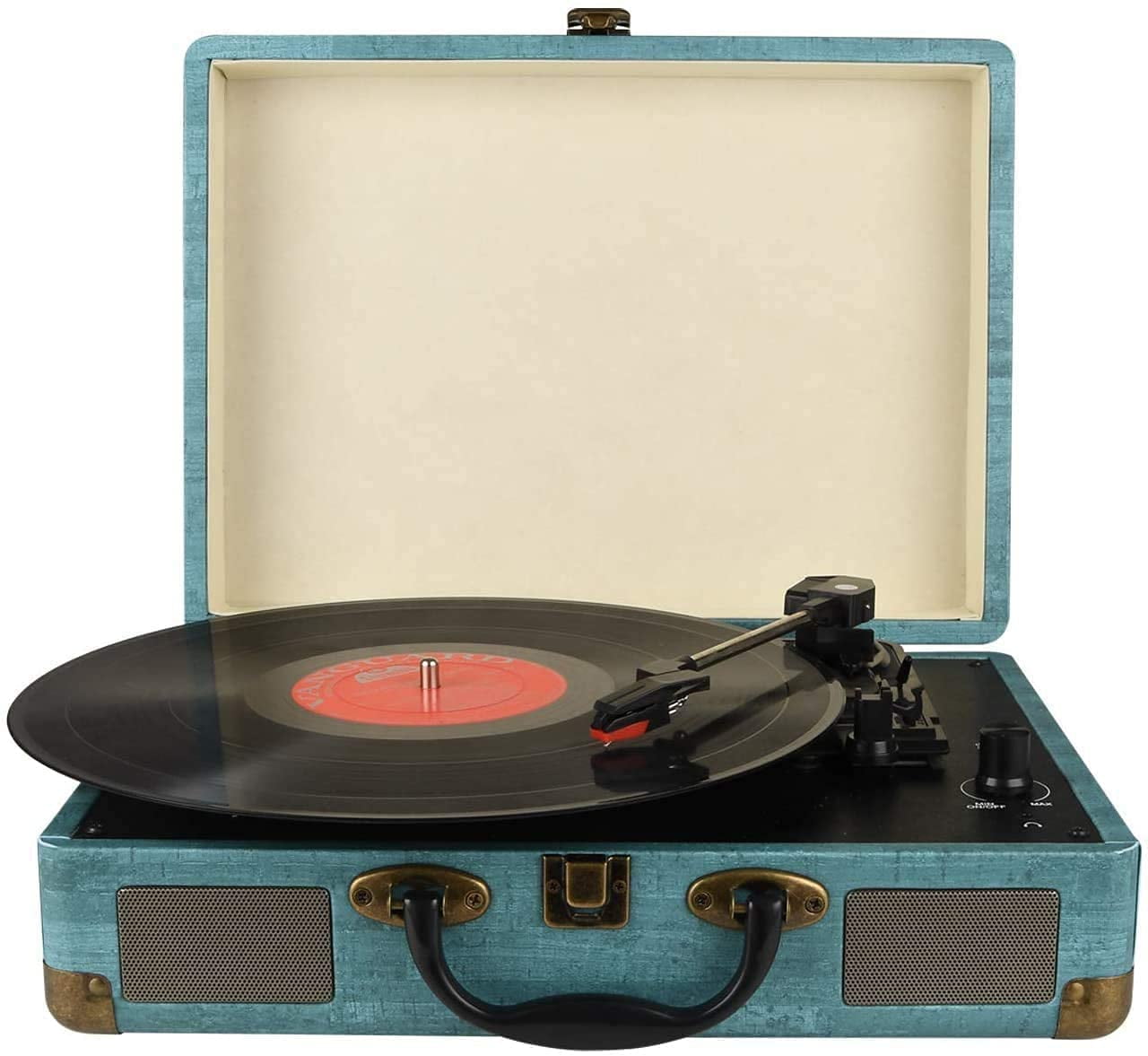This color photograph showcases an old-fashioned record player from the 1950s or 60s, designed to resemble a medium blue suitcase with a front handle and two gray speaker vents on either side. The suitcase's lid is open, revealing a cream-colored interior, and a black latch and corner fittings in brass or gold add vintage charm. The record player is actively playing a vinyl record, with the black armature halfway through the spinning disc. The record features a red inner label and is anchored by a silver peg. Alongside the turntable mechanism, there are a couple of knobs for adjustments.